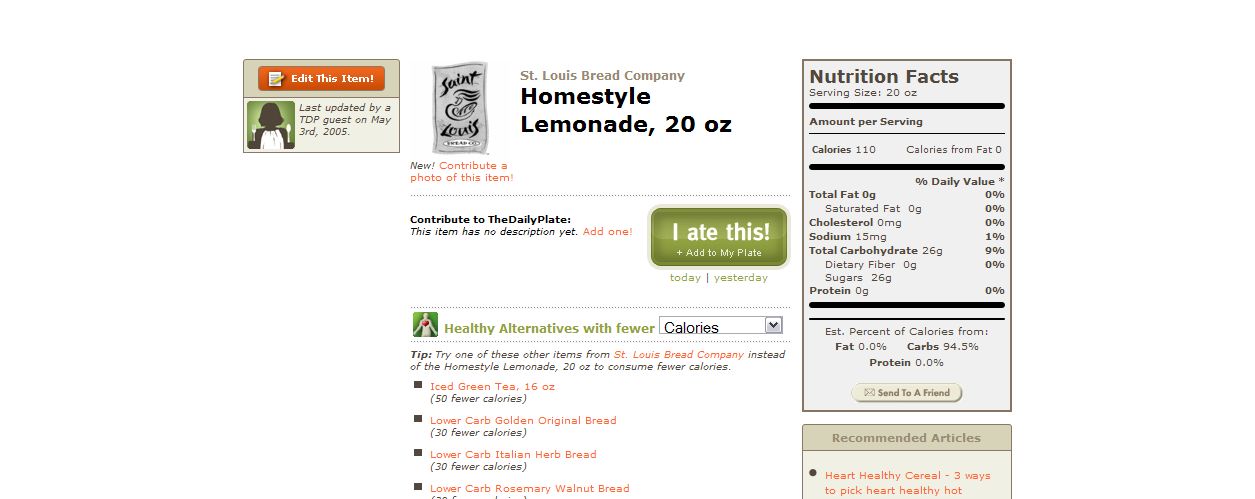The image depicts a website design layout focused on nutrition and healthy eating. 

In the top left corner, there's a header reading "Edited Site," with a subheadline stating "Last updated by a TD (guest?) on May 2nd, 2005." To the right, the site prominently features the "St. Louis Bread Company" alongside an item titled "Homestyle Lemonade," which is specified as coming in a 20-ounce serving. A phrase below this section reads, "Contribute to the daily plate."

A green square below the header contains the text "I eat this," followed by a suggestion to explore "Healthy alternatives with fewer calories" through a dropdown menu. The site recommends trying other items from St. Louis Bread Company instead of the Homestyle Lemonade, such as ice cream or tea in a 16-ounce serving that has 50 fewer calories and lower carbs. Additional items suggested include "Golden Original" and "Rosemary Walnut Bread."

A nutrition facts label is located in the top right corner, providing detailed nutritional information for the selected food item. The bottom right corner highlights recommended articles with titles like "Heart Healthy Cereal" and "Three Ways to Pick Heart Healthy."

Above these recommended articles, there's a call-to-action with the text "Email to a friend," followed by some descriptive content.